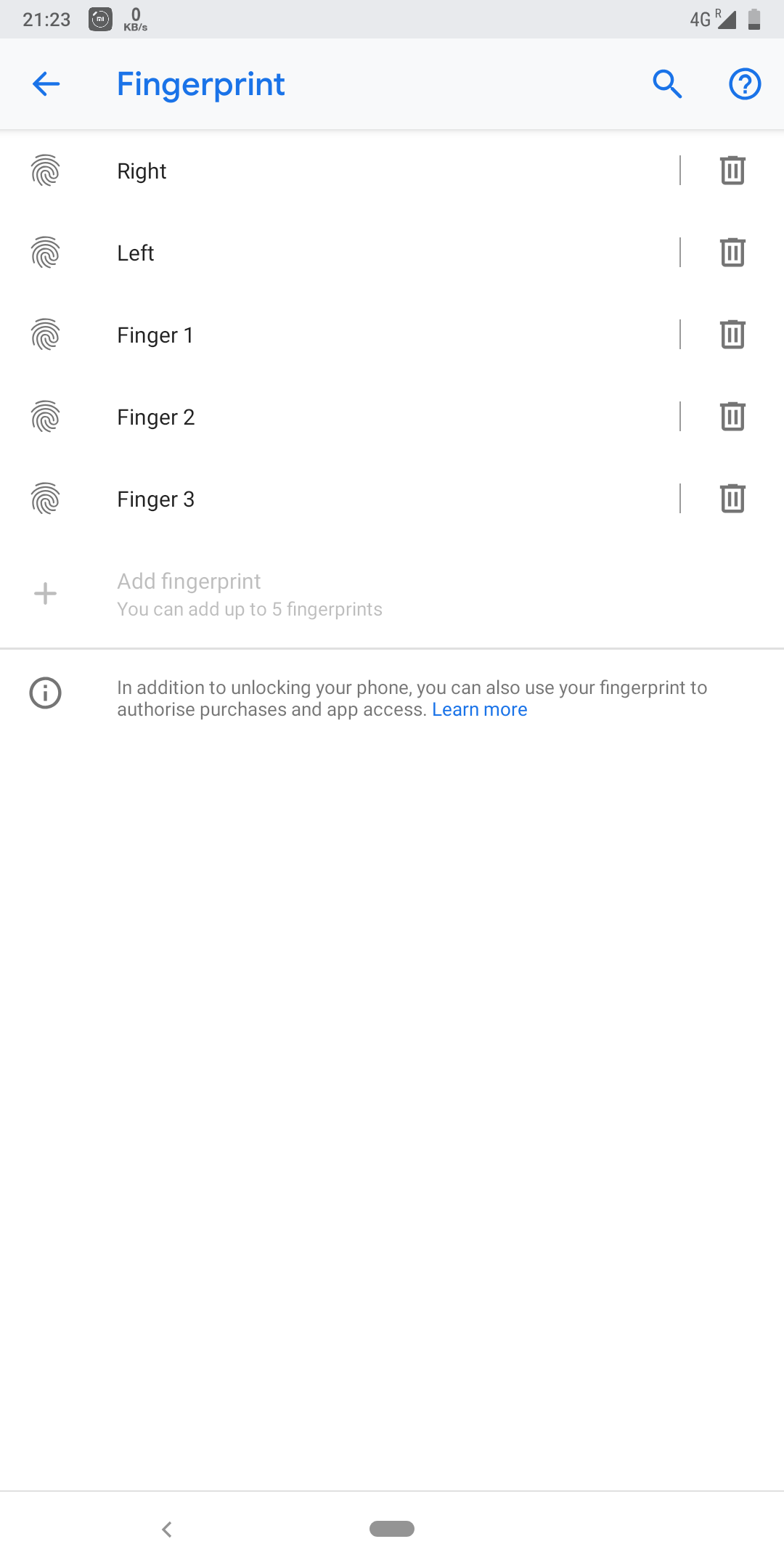The image depicts a partial view of a cell phone screen. At the top left corner, the time is displayed as 21:23. The top right corner contains a signal strength icon and a battery icon showing approximately 25% charge, both against a light gray background. The rest of the screen's background is white.

Directly below the top bar, in blue text, is the word "Fingerprint." To its left is a blue arrow pointing left, and to its right are a search icon and a small circle with a question mark inside. 

Beneath this section, there are five categories arranged vertically: "Right," "Left," "Finger 1," "Finger 2," and "Finger 3." Each category has a small icon to its left, a small vertical line, and a trash can icon on its right. 

At the bottom of this list is an option labeled "Add fingerprint," accompanied by small gray text that states, "You can add up to five fingerprints." A plus sign is positioned to the left of this text. Below this, a horizontal line separates the content from a final icon that features a black sentence followed by blue text reading "Learn more."